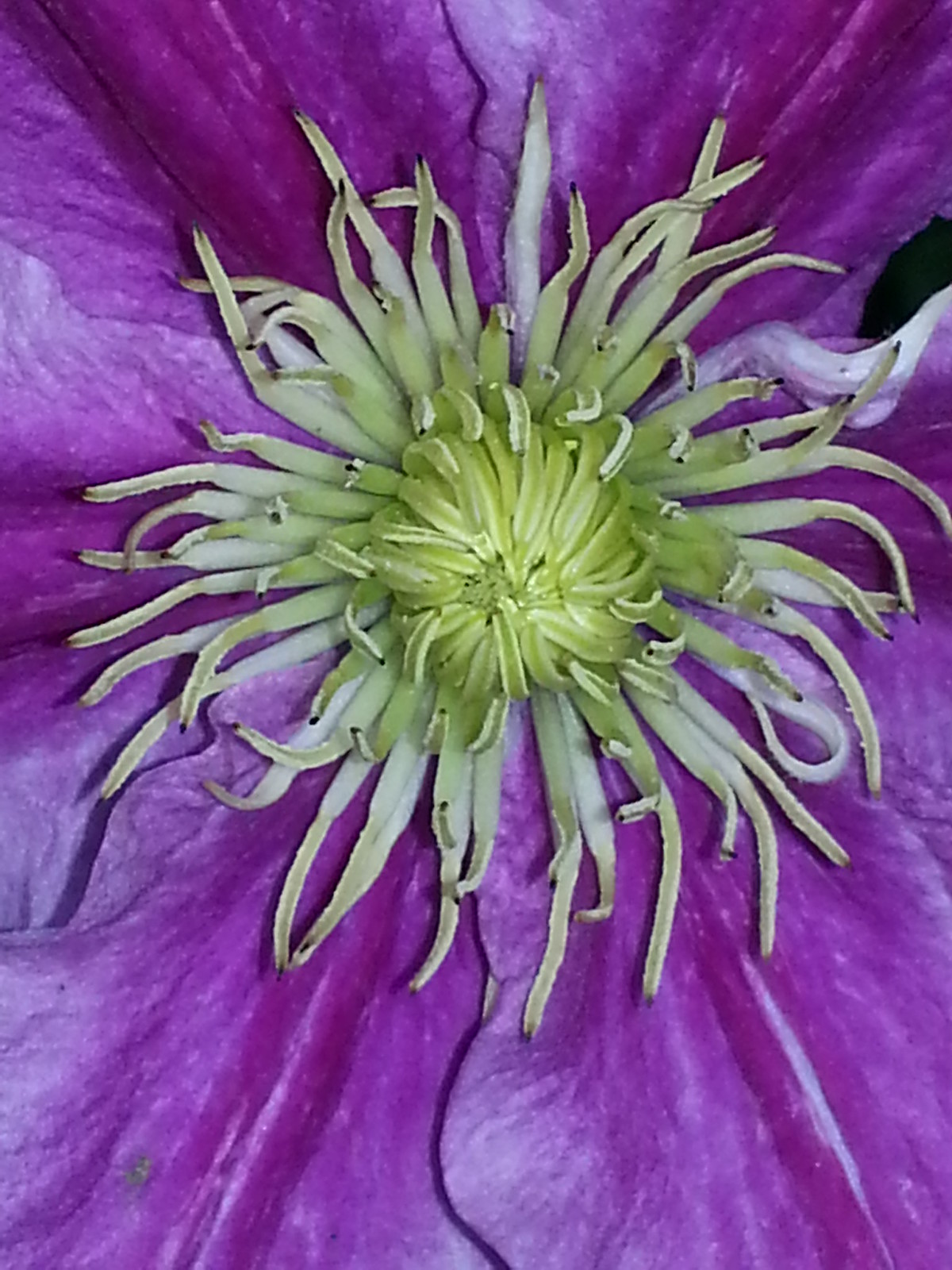The image captures an intimate close-up of a pansy flower in mid-bloom, prominently showcasing its central pistil. The pistil, featuring shades of bright green and white with a delicate feathery structure, stands out against the vibrant violet petals that envelop it. These petals exhibit a dynamic range of colors, transitioning from deep to lighter purples, and include delicate, curled edges that frame the central structure. Some petals even show a gradient to nearly white at their brightest points. The flower's layout reveals layers radiating outward from the pistil, with the very center seemingly more clustered and unopened, like a pod, indicating the flower hasn’t fully bloomed yet. The image seems to be taken at nighttime, as suggested by the dark, almost black background visible in the upper right corner, adding a striking contrast to the vivid colors of the petals and pistil.